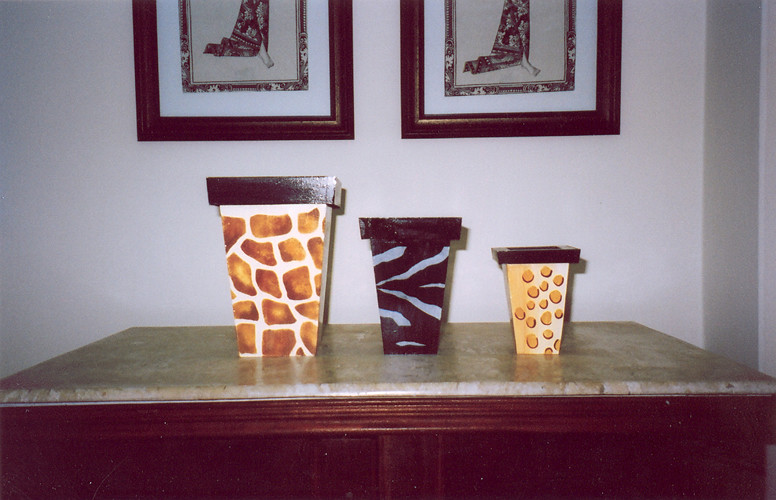The image depicts a straight-on view of a hallway accent table crafted from dark brown wood, topped with a tan marble surface. Atop the marble surface are three decorative vases of descending size from left to right. Each vase features a square base with dark brown top edges. The largest vase on the left has a tan background adorned with brown spots that resemble a giraffe's skin. The central vase, medium in size, showcases a dark brown background with off-gray diagonal stripes mimicking zebra-like patterns. The smallest vase on the right has a tan background with darker tan dots suggestive of cheetah spots. These animal-themed vases are positioned against a white wall, above which hang two identical framed images in dark brown frames. The images appear to depict antique-style art, possibly featuring oriental motifs. The entire setup suggests a blend of artistic elegance and exotic animal prints, harmoniously arranged on a stylish piece of furniture.